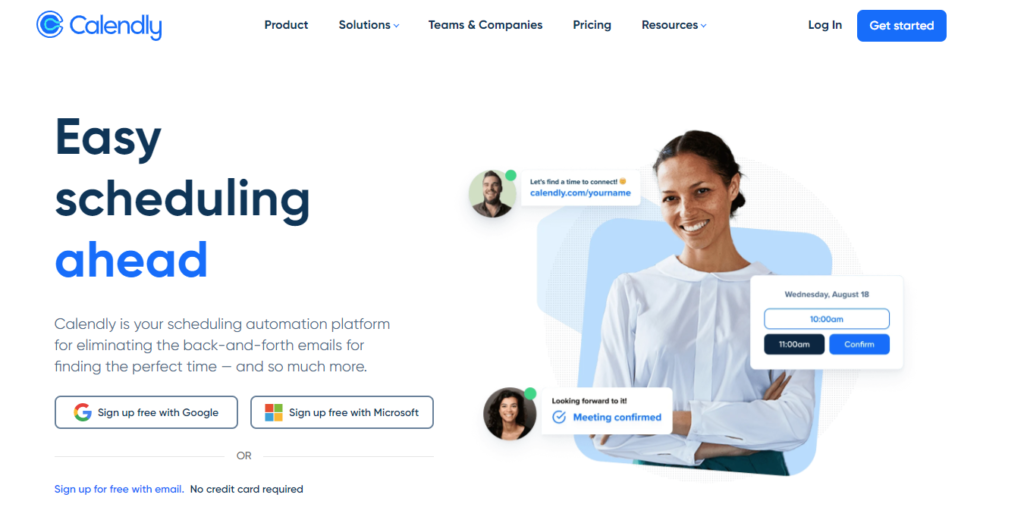Screenshot of Calendly's Homepage:

At the top left corner of the page is the Calendly logo, consisting of the word "Calendly" in blue text, accompanied by a blue and white "C" emblem to its left. The navigation menu spans the top section of the page, featuring the options: Product, Solutions, Teams and Companies, Pricing, and Resources. Towards the right of the menu, there are two links: "Login" and a prominent blue "Get Started" button.

Dominating the center of the page is a large header section with the text "Easy Scheduling Ahead" in blue. Below this, a subheader reads: "Calendly is your scheduling automation platform for eliminating the back and forth emails for finding the perfect time, and so much more."

Beneath the subheader, there are two sign-up buttons: "Sign up free with Google" on the left, adorned with the Google logo, and "Sign up free with Microsoft" on the right, featuring the Microsoft logo.